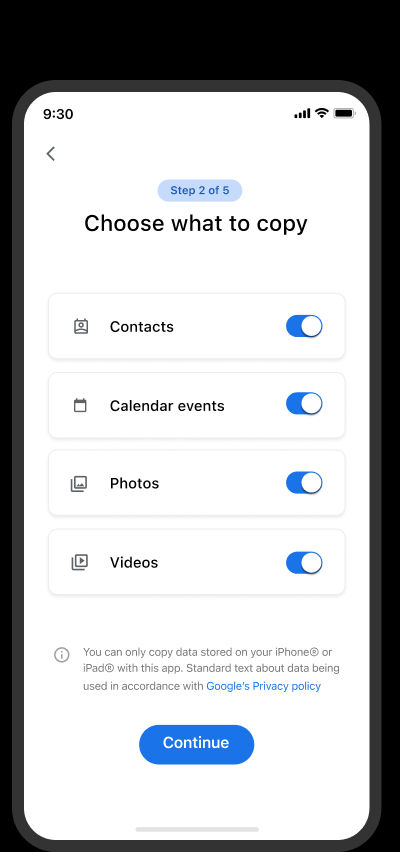This image is a detailed screenshot of a settings page on a mobile phone. At the top of the screen, there's a black arrow pointing left, indicating a back button. Next to it, within a blue pill-shaped area, the text "Step 2 of 5" is prominently displayed. Below this header, there's a prompt that reads "Choose what to copy."

Four options are presented in vertically aligned boxes just below the prompt, each containing an icon on the left, descriptive text in the middle, and a blue toggle button on the right. The options available for selection are:
- Contacts
- Calendar events
- Photos
- Videos

Each of these options has the toggle button set to the "on" position. At the bottom of this section, a note informs users that only data stored on their iPhone or iPad can be copied using this app. There's also standard text regarding the usage of data in accordance with Google's privacy policy. Finally, a blue pill-shaped "Continue" button is located at the very bottom of the screen. The phone is displayed against a black background, which emphasizes the interface of the mobile device.